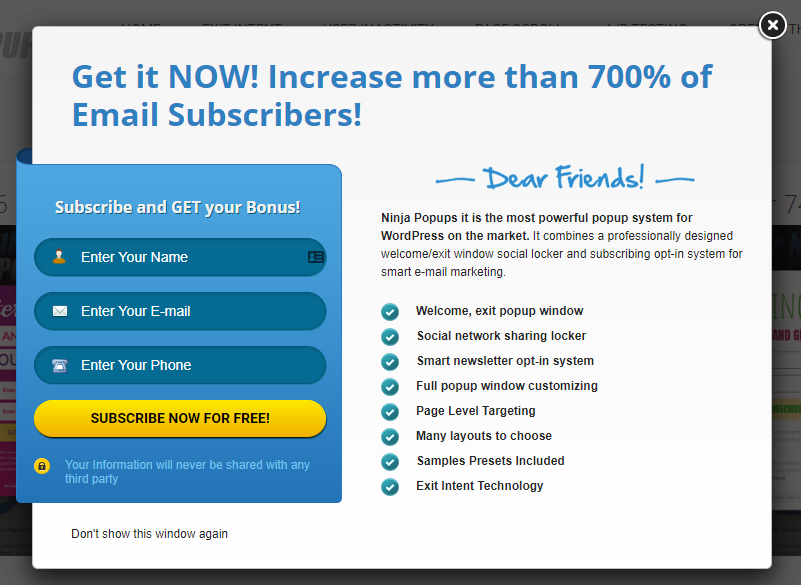This image appears to be an advertisement from a website, indicated by a black border with a small white X in a circular black icon in the upper right corner, suggesting it can be clicked to close the ad. The central background is white, prominently featuring a call-to-action in bold text at the top that reads, "Get it now, increase more than 700% of email subscribers."

Underneath this headline, in elegant blue script, it addresses, "Dear Friends," followed by detailed messaging in black text stating, "Ninja Pop-Ups is the most powerful pop-up system for WordPress on the market. It combines a professionally designed welcome/exit window, social locker, and subscribing opt-in system for smart email marketing." 

Below this description, a series of benefits are listed with blue check marks, highlighting features such as a welcome exit popup window and social network sharing locker. On the left-hand side of the image, a blue box with the prompt, "Subscribe and get your bonus," invites users to enter their name, email, and phone number. A yellow horizontal oval below this input form reads, "Subscribe now for free."

Additionally, a note below the form reassures that user information will never be shared with any third party, and an option, "Don't show this window again," is also provided. The ad is well-structured to engage users with a clear, step-by-step subscription process and emphasizes the security and benefits of subscribing.